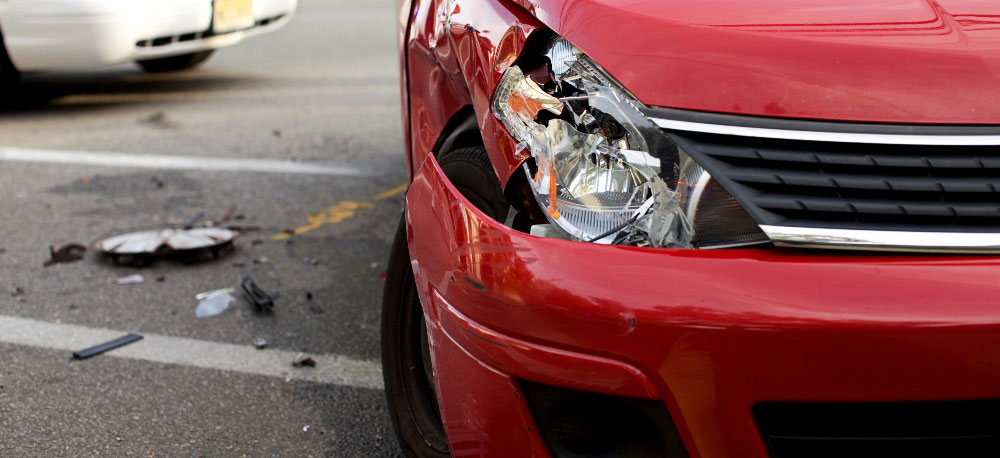The image captures a close-up of a red car's front left side, clearly damaged from an accident. The bumper is scratched and dented, focusing on the headlight area, which is smashed. The broken front fender and a slightly damaged passenger side door are visible, along with a hubcap and various black fragments scattered on the pavement. Positioned on asphalt marked with two white parking lines, the scene suggests it took place in a parking lot. In the background, the rear end of a white car is barely visible, possibly hinting at its involvement in the accident.